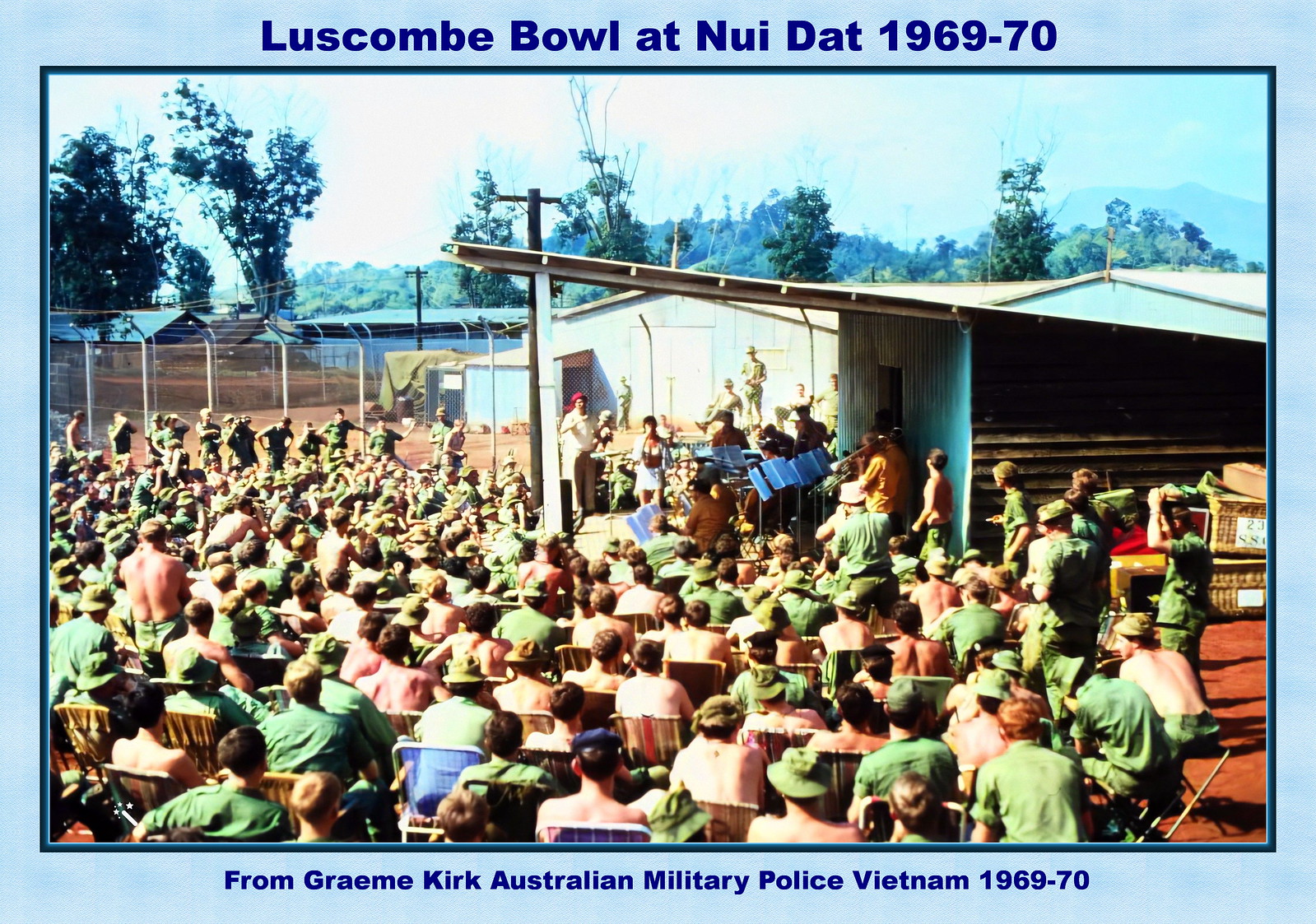The image captures a lively scene at a military camp outdoor concert, likely around 1969-1970. Soldiers, roughly half shirtless and half in full green uniforms, are seated on large chairs, attentively watching the performance. The backdrop includes a fence, several shacks, buildings, trees, hills, and a clear sky. At the forefront under a house's roof or possibly a metal building overhang, a female singer, a conductor, and a sizable band are positioned. Band members are engaged with sheet music, playing various instruments such as trumpets and trombones. The photo features a blue border with captions reading "Luscombe Bowl at Nui Dat, 1969-1970" at the top and "From Graham Kirk, Australian Military Police, Vietnam, 1969-1970" at the bottom. The audience appears engrossed in the musical performance, embodying a moment of communal respite and entertainment amid their service.